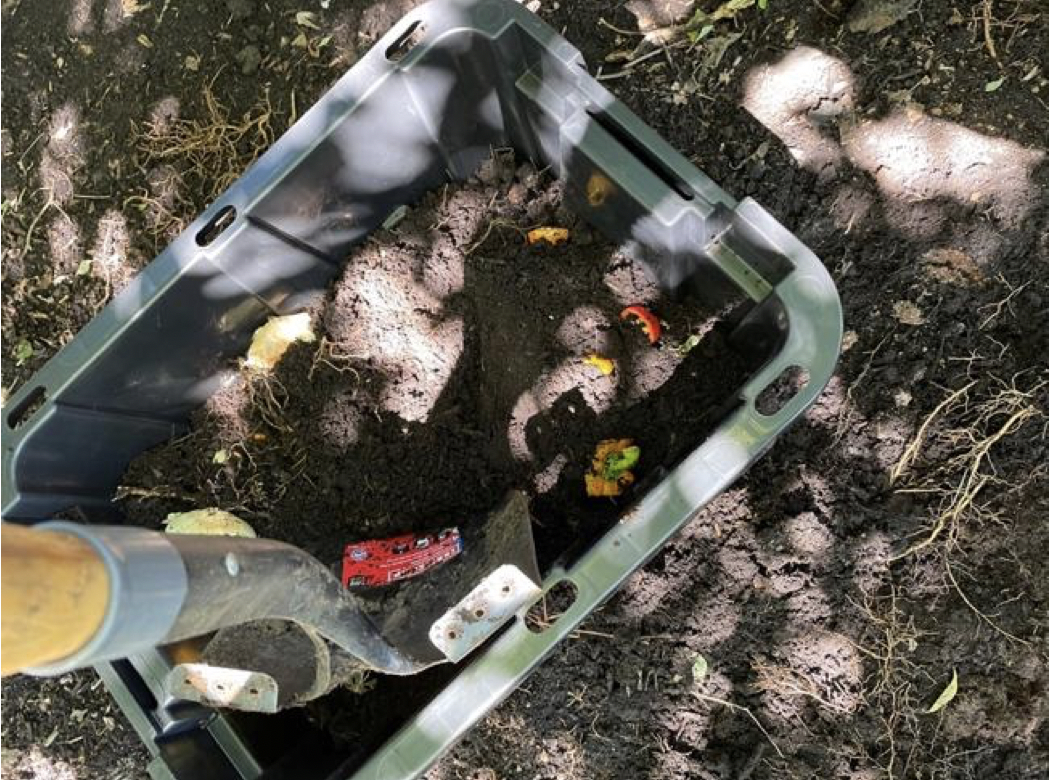This image captures an outdoor garden scene characterized by an abundance of dirt and weeds in the background. At the center, there is a large gray plastic container filled with soil and various indistinct objects, one of which appears to be a tomato. A shovel, captured from above, is seen plunging into the container, revealing both its wooden handle and the metal blade. The blade still retains a red, unreadable label, adding a touch of color to the otherwise muted tones of the garden. The background hints at freshly disturbed earth, suggesting the early stages of a gardening project. No visible plants emerge from the soil, indicating that this might be preparation work for future planting. The image, though slightly out of focus, conveys the essence of a gardener's preliminary efforts in readying the plot for the coming season.